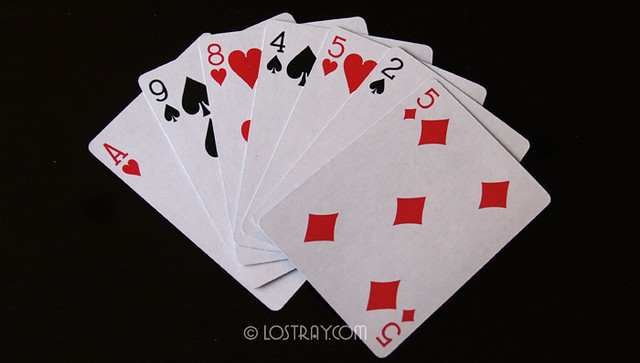The image is a rectangular photograph with the longer sides extending horizontally. The backdrop is completely black, creating a stark contrast for the main subject. At the bottom center of the image, there is a small, white watermark with the text "© lostray.com."

The focal point of the image is a fan-like spread of seven playing cards, meticulously laid out from left to right. The far left card is the Ace of Hearts, angled towards the upper left corner. Next, the Nine of Spades is slightly more upright but still leaning left. Following that, the Eight of Hearts stands even more upright. The sequence continues with the Four of Spades, which begins to tilt slightly to the right. Subsequent to that is the Five of Hearts, leaning further to the right. Then comes the Two of Spades, pointing more rightward. Finally, the sequence ends with the Five of Diamonds, which points sharply towards the right corner. Notably, the cards alternate in color between red and black, enhancing the visual appeal and organization of the layout.